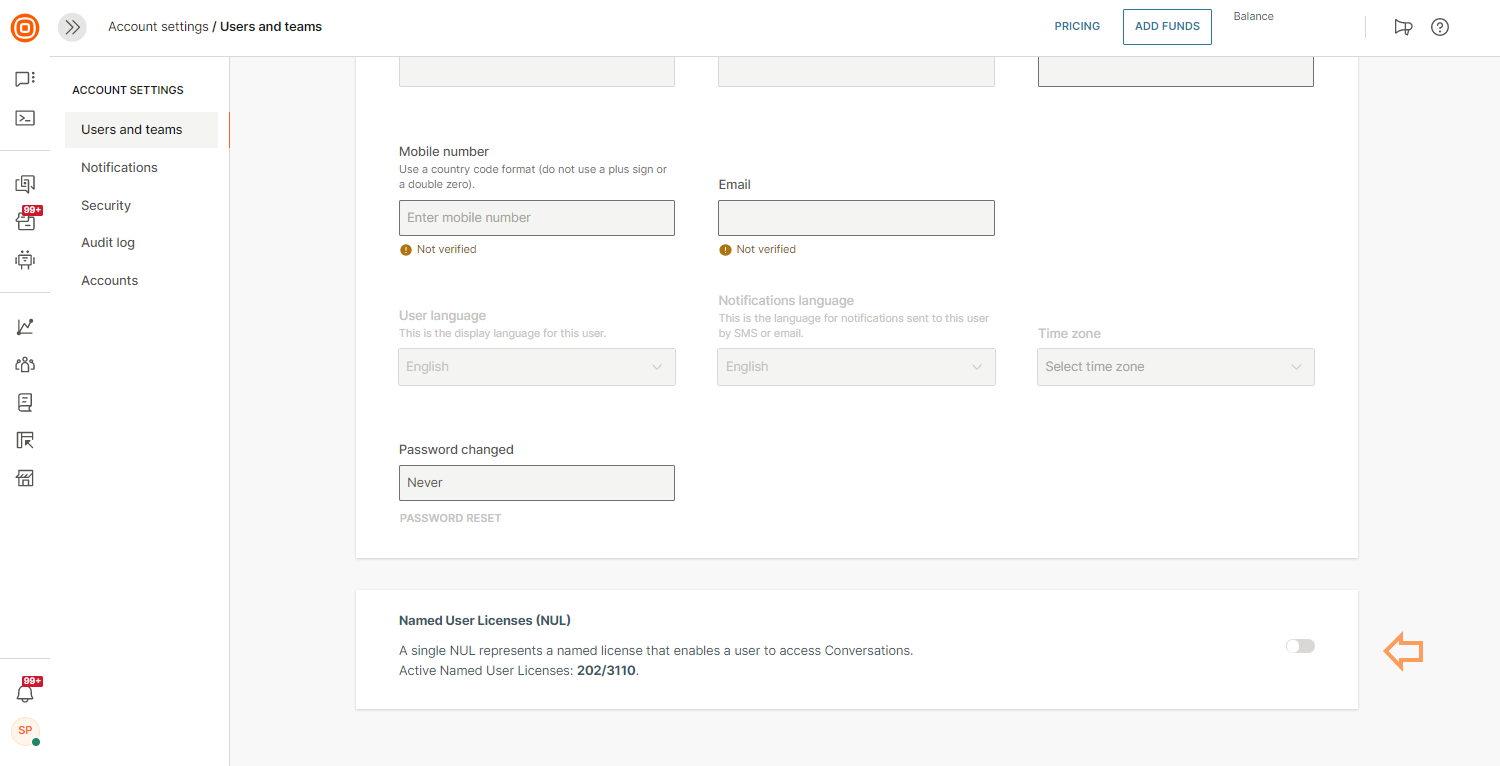This screenshot captures the "Account Settings: Users and Teams" page within a computer application or website. 

In the top left-hand corner, an orange bullseye icon is prominently displayed, followed by a gray right-pointing arrow. Adjacent to the arrow, the text reads "Account Settings / Users and Teams." 

In the top right-hand corner, a "Pricing" button is visible in blue font. Nearby, a button with a blue border displays options to "Add Funds." Below this, a gray font indicates your account "Balance."

On the left side of the screen, there is a navigational menu featuring different categories. The currently selected category is "Users and Teams," and the menu options beneath include "Notification," "Security," "Audit Log," and "Accounts." Further left, there is a vertical row of icons to access additional menus.

The main screen area has a gray background with several white boxes overlaying it. These white boxes contain personal information fields. At the top, the label "Mobile Number" appears with two text boxes below. Another section is labeled "Password Change" with a status box below indicating "Never."

Towards the bottom right corner of the screen, an orange arrow points to a white box labeled "Named User Licenses."